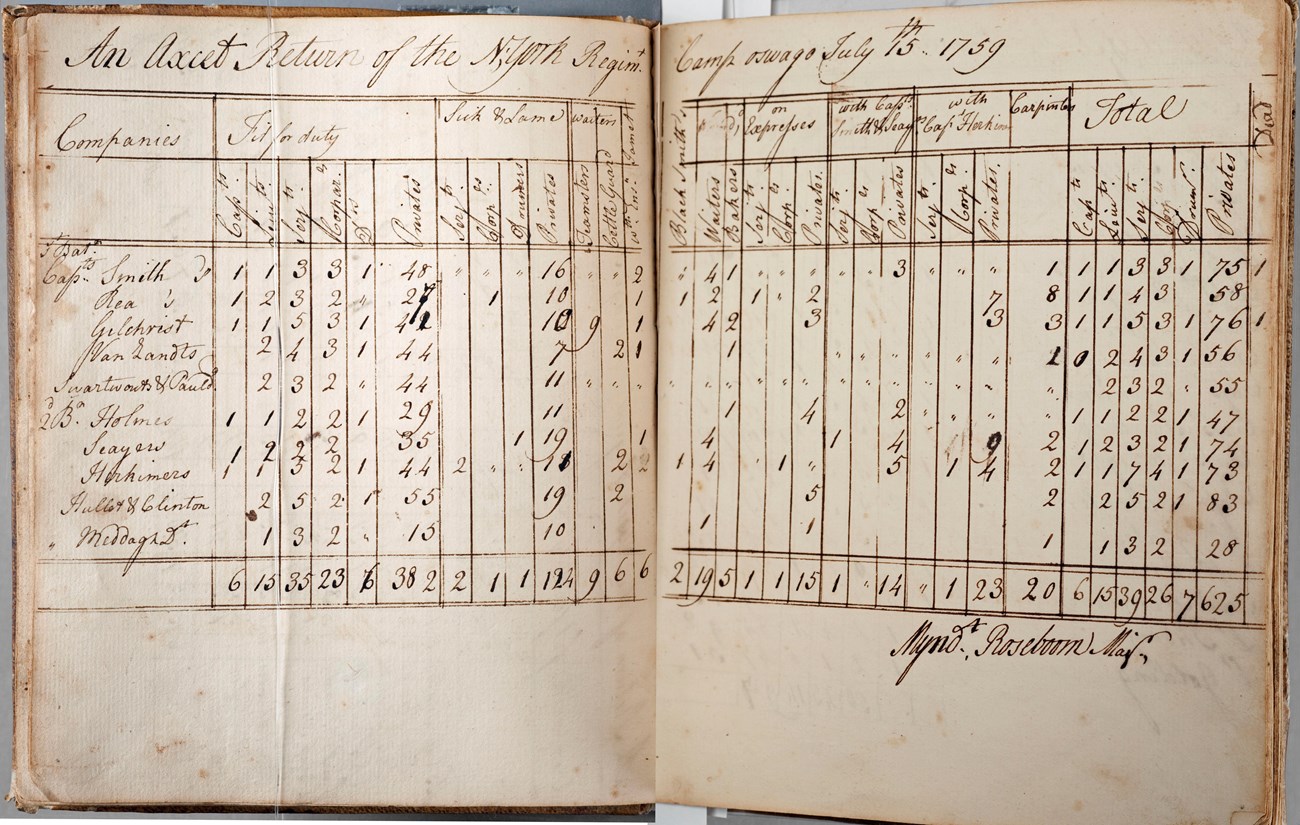This image captures an ancient, open notebook that appears to be a ship's log, dating back to July 15, 1759. The aged pages are filled with cursive handwriting that is difficult to decipher, indicating its antiquity. The spread shows detailed charts with columns and rows, seemingly used for bookkeeping purposes, listing various companies in the far-left column and totals in the far-right column. The brownish text and numerous smudges further accentuate the notebook's old-fashioned and worn-out appearance. This artifact provides a glimpse into historical maritime record-keeping practices, reflecting its status as a relic from a bygone era.